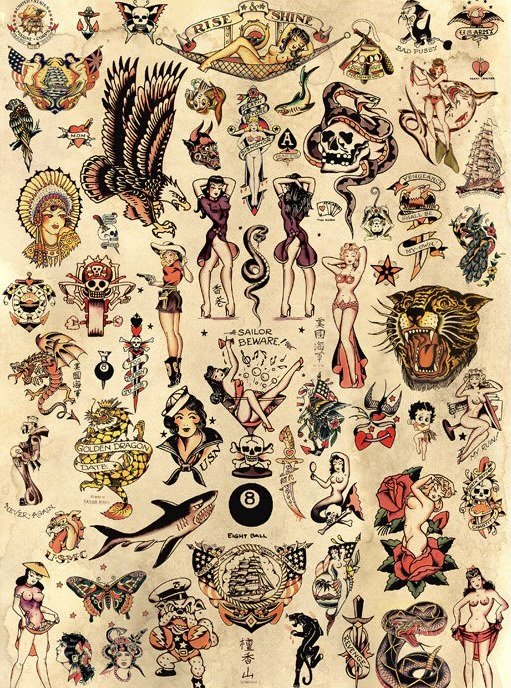This is a vertically aligned, hand-drawn poster set against a beige (light tan) background, densely packed with a multitude of colorful illustrations, predominantly of women in various stages of dress and undress. The image features a banner at the top proclaiming, "Rise and Shine," beneath which a nude woman reclines in a hammock with flowers over her upturned knee. Surrounding her are a myriad of small, detailed drawings, including:

- Various women in different postures and attire, often nude or partially clad, such as a woman wearing a cowboy hat and short shorts holding a gun, a bikini-clad woman with a robe behind her, and a woman with a sailor's cap and "U.S. Navy" dress.
- Numerous animals such as an eagle with its wings raised and an angry expression, a large snarling tiger's face, a bulldog wearing a sailor's cap, a snake, and a butterfly.
- Several icons and symbols like a skull and crossbones, a sailboat, an eight-ball, a dragon labeled "Golden Dragon Date," and a skull on a flag.
- Additional quirky details such as a woman inside a cocktail glass with "Sailor, Beware of Buffalo" written below, a cat with "Bad Pussy" underneath, and a lizard.

The poster includes scattered, selective color elements, with deep reds, blacks, purples, and some blues, especially in the details of the various figures and objects. A man with Popeye-like bulked-up arms, an ornate Indian chief headdress, and a character resembling Betty Boop also make appearances. Various flags, including the American and UK flags, add to the chaotic but intricate tapestry of this hand-drawn artwork.